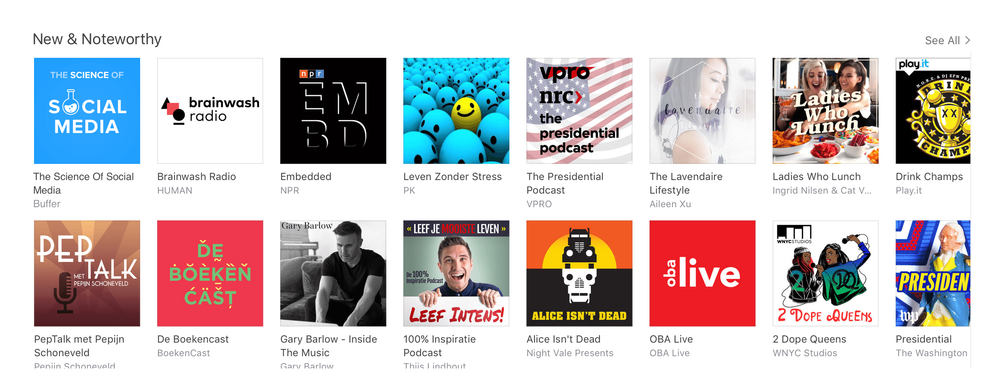In the upper left-hand corner of this image, a label reads "New and Noteworthy." The image showcases two horizontal rows, each containing eight items under this label. To the right side of the display, there is an option that says "See All."

In the top row, starting from the left, the items are as follows:
1. The Science of Social Media
2. Brainwash Radio
3. Embedded
4. Legends Under Stress
5. The Presidential Podcast
6. The Lavender Lifestyle
7. Ladies Who Lunch
8. Drink Champs

In the bottom row, beginning from the left, the items are:
1. Pep Talk
2. Dr. Deboeken
3. Gary Barlow
4. 100% and Spurt Podcast
5. Alice Isn't Dead

The image is a curated list highlighting notable new podcasts or shows, providing a snapshot of popular or trending content.